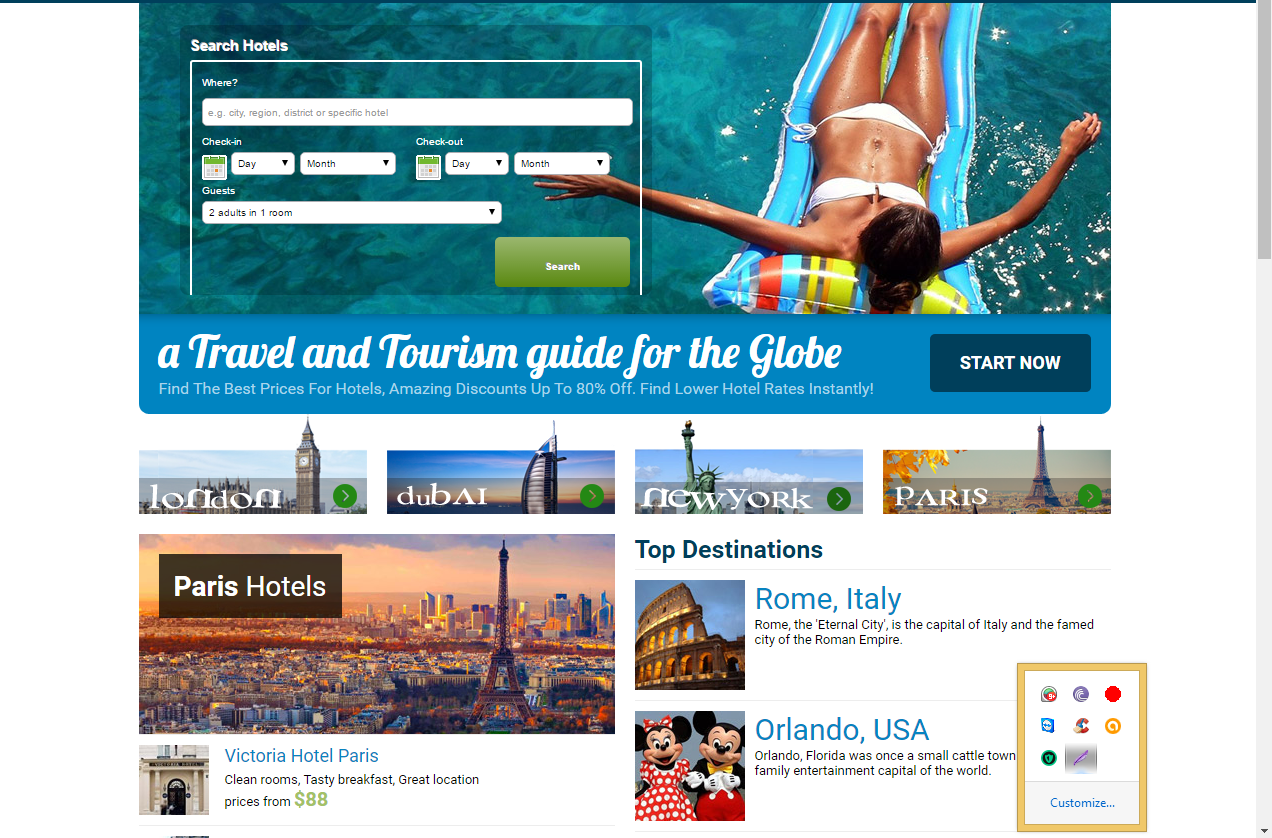**Detailed Caption:**

The web page features a visually striking image showcasing a tranquil cyan-blue water body with darker blue tones interspersed within it. A woman with an olive complexion lays relaxed on a floating bed. She is clad in a two-piece white bikini and her black hair, which appears to be at least shoulder-length, is styled in a bun. The floatation device she is on has vibrant strap stripes in cyan blue, red, green, forest green, and orange.

To the left of the image is a search section with a large rectangular area at the top stating "Search Hotels" in white text. Below this, a white rectangle is provided for entering the destination. Adjacent to the destination input are two green and white calendars labeled "Check-in" and "Check-out," each with drop-down menus for selecting the day and month. Below these calendars is a section to specify guests, with a default example showing "2 adults in 1 room," which can be adjusted via a drop-down menu. To the right, within the same rectangle, there is a dark green button that reads "Search" in white text.

Surrounding this search section is a bezel outlined in dark blue, containing bold white text that reads, "A Travel and Tourism Guide for the Globe." Below this heading, in thinner white text, the page advertises: "Find the best prices for hotels, amazing discounts up to 80%! Find lower hotel rates instantly!"

On the right-hand side, a dark blue button features bold white text stating "Start Now."

The central section showcases iconic travel destinations with images: London with the London Tower, Dubai with its famous tower, New York with the Statue of Liberty, and Paris with the Eiffel Tower. 

Towards the lower left of the page, an aerial view of Paris is labeled "Paris Hotels" in bold white, accompanied by details about the city. The text explains, in hyperlink blue, the top destinations like the Roman Colosseum paired with "Rome, Italy," and a brief description of Rome as "The Eternal City and the capital of Italy and the famed city of the Roman Empire." 

Additionally, the page features an image of Mickey and Minnie Mouse, labeled "Orlando, USA" in hyperlink blue text. Below this, a short description reads: "Orlando, Florida was once a small cattle town and is now the family entertainment capital of the world."